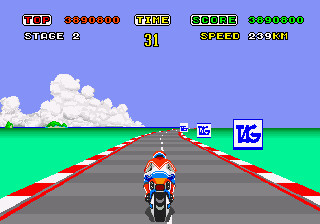This small, square screenshot features an 8 or 16-bit video game from the 1980s or 1990s, showcasing a motorcycle racing scene. The main focus is a pixelated motorcycle rider dressed in a red and white jacket with blue pants, red boots, and a red helmet with white and blue stripes. The motorcycle, with an orange seat and a visible black back wheel, rides down the center of a two-lane grey road, which alternates between dark and light shades. The sides of the road are bordered by alternating red and white stripes, indicating the out-of-bounds area, and beyond those stripes lies a stretch of green grass. In the background, a blue sky with cloud coverage in the bottom left corner and distant trees can be seen. On the right side of the road, white signs with blue borders and the word "TAG" in blue lettering are spaced along the edge. The top of the screen displays various game statistics, including "Stage 2" in white, the player's top score in red, playtime, total score, and the motorcycle's speed, all rendered in the game's retro pixelated art style.